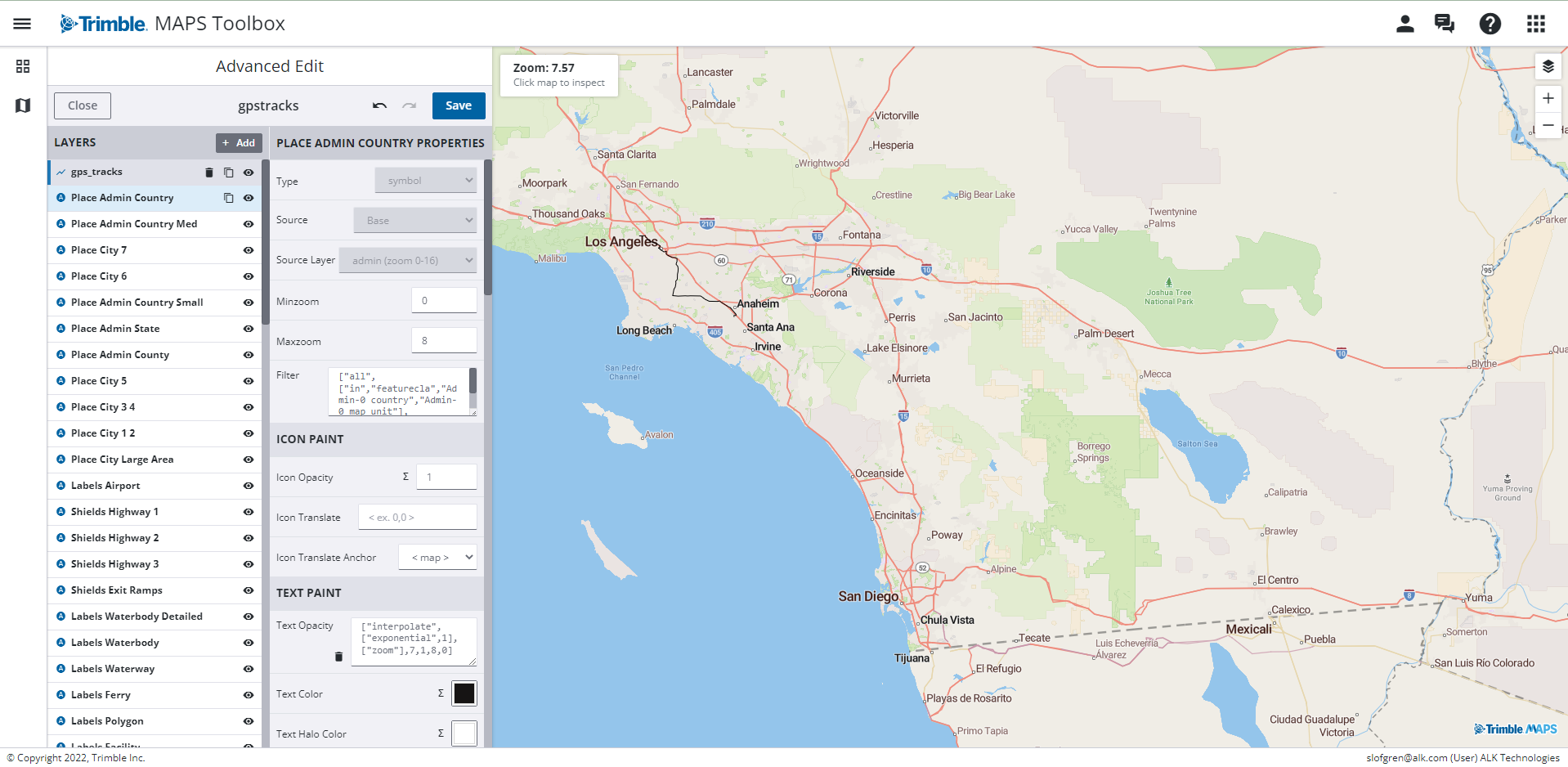The image is a screenshot of the Trimble Maps Toolbox interface. Dominating the right side of the screen is a detailed map reminiscent of a Google Maps layout, focusing on the Southern California region, including Los Angeles and San Diego. The map is populated with various highway markers and symbols, although the specifics are not easily readable. On the left side, there are two scrollable panes designed for adding, removing, and editing map elements. The Trimble Maps Toolbox branding is prominently displayed in blue. Additional interface features include a person icon, chat support, a help question mark, and a hamburger menu located on the far right. Additionally, plus and minus symbols for map zoom functionality are present. The ocean and the sprawling Greater Los Angeles area are noticeably represented on the map.